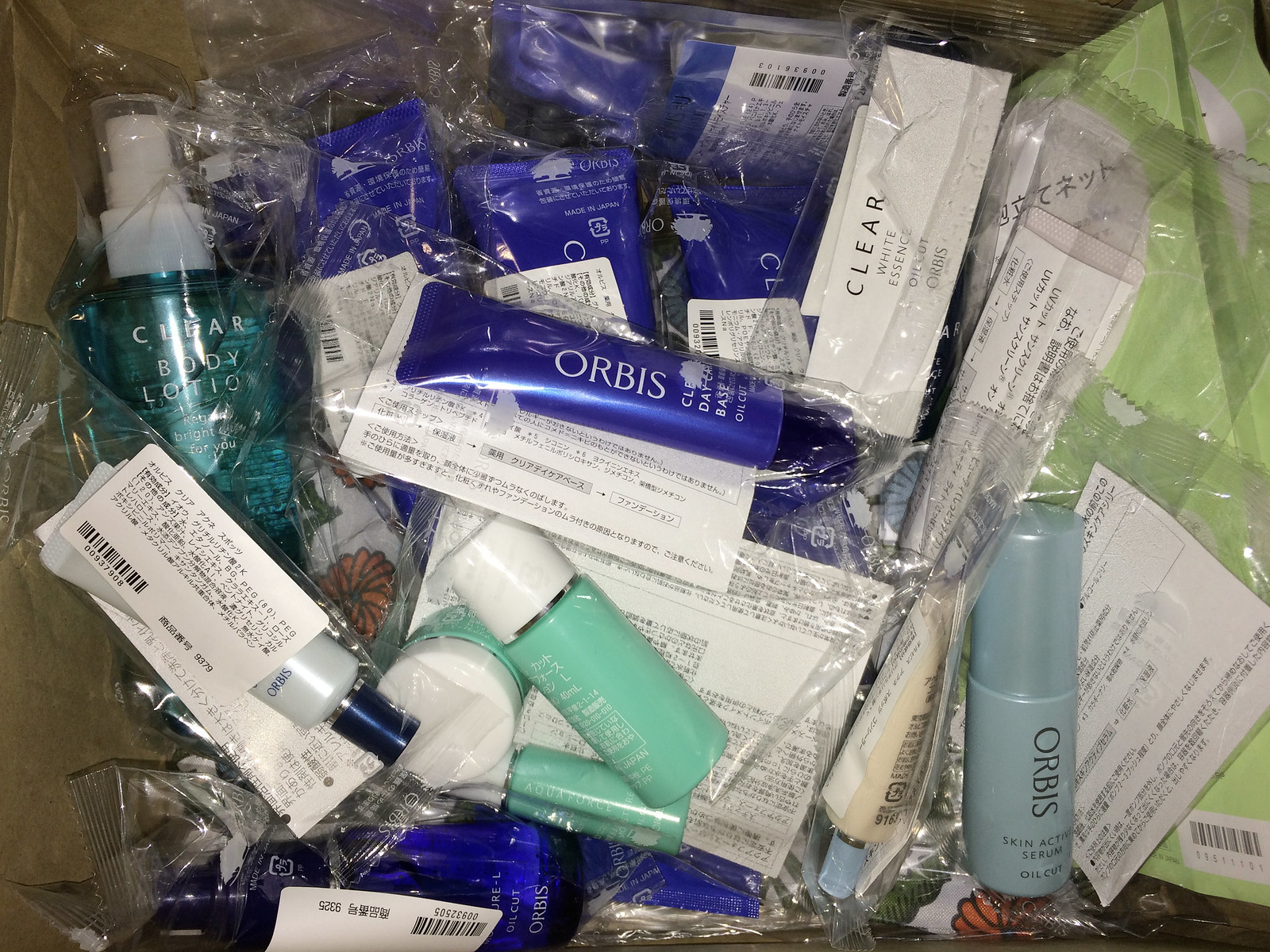A pile of individually sealed Japanese cosmetics, predominantly featuring the Orbis brand, is jumbled together. Each product is encased in a clear plastic cellophane wrapper, making it challenging to discern specific items due to glare. The packaging includes Japanese text, likely indicating product details. Notable items in the pile include a blue-labeled Orbis squeeze tube with a partially visible 'day base' label, and a small cylindrical bottle marked as Orbis' 'skin active serum, oil cut.' Other visible labels mention 'clear white essence' and 'something oil.' The products are arranged haphazardly, suggesting a collection of various Orbis cosmetics.